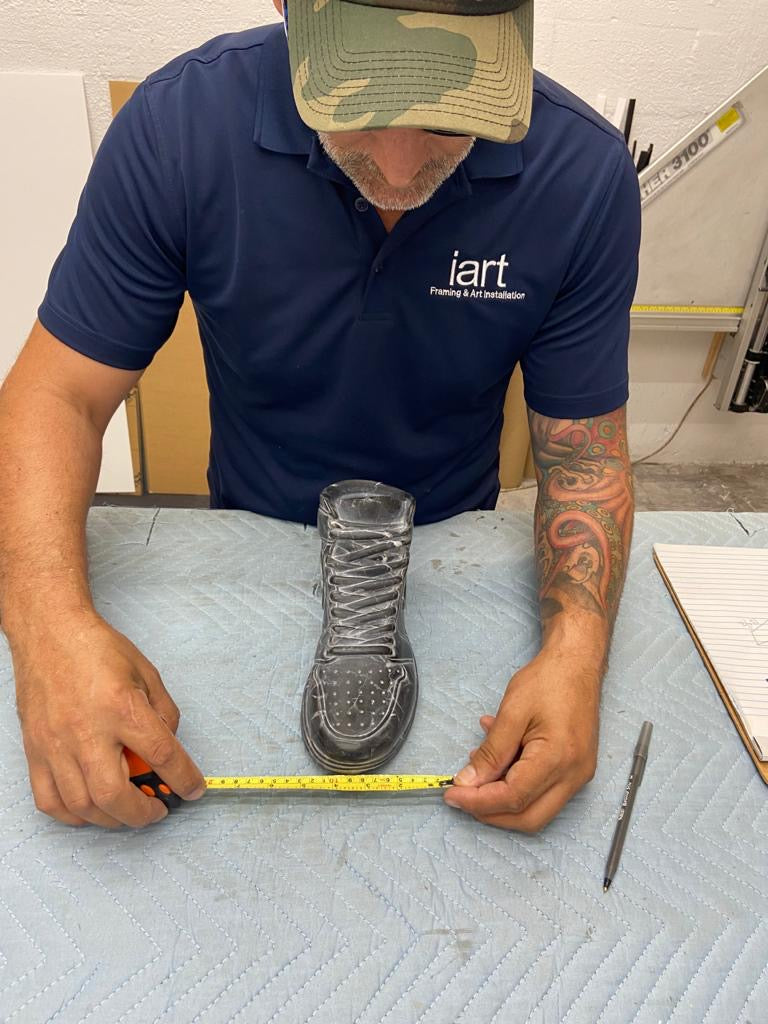The image is a detailed color photograph depicting a man, likely a museum conservator or an artist, meticulously measuring a shoe sculpture with a measuring tape. The shoe, which appears to be an intricate bronze or dark gray cast artwork, is centrally placed on a light blue quilted mat typically used for protecting fragile items. The man, donning a green camouflage baseball cap, sports a short stubbly beard with a hint of gray and is dressed in a blue shirt emblazoned with the text "I heart, I art." His left arm, detailed with tattoos, rests near a small ballpoint pen and an opened clipboard or piece of paper. In the background, a white brick wall adorned with measuring or framing equipment can be seen, suggesting a workshop or studio environment.